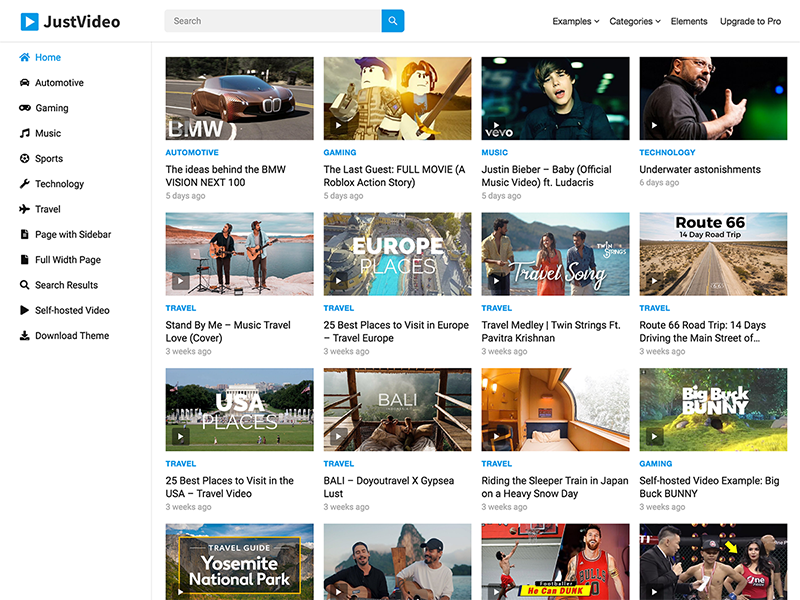This is a cropped screenshot of the webpage "Just Video". The background of the webpage is white. At the top left corner, the "Just Video" logo is prominently displayed. Adjacent to the logo on the right is a search bar. Further to the right are navigation links labeled "Examples", "Categories", "Elements", and "Upgrade to Pro".

Directly beneath this top navigation section, a sidebar column on the left lists various categories: Home, Automotive, Gaming, Music, Sports, Technology, Travel, Page with Sidebar, Page with Full Width Page, Search Results, Self-hosted Videos, and Download Theme. The category "Page with Sidebar" is currently selected.

The main content area to the right of the sidebar features an array of video thumbnails organized into a grid layout. Each row contains four video thumbnails, making a total of four fully visible rows on the page. 

In the first row, the thumbnail on the far left depicts a futuristic BMW under the category "Automotive," highlighted in blue in the upper left corner of the thumbnail. Below the thumbnail, the title of the video is displayed, followed by the upload time "five days ago."

To the right of this automotive video, there is a gaming video featuring Roblox characters. The category "Gaming" is marked in the upper left corner, and the video's title is "The Last Guest: A Roblox Action Story."

The page continues to display various video thumbnails, showcasing a broad spectrum of interests and categories, making it a comprehensive space for video exploration.